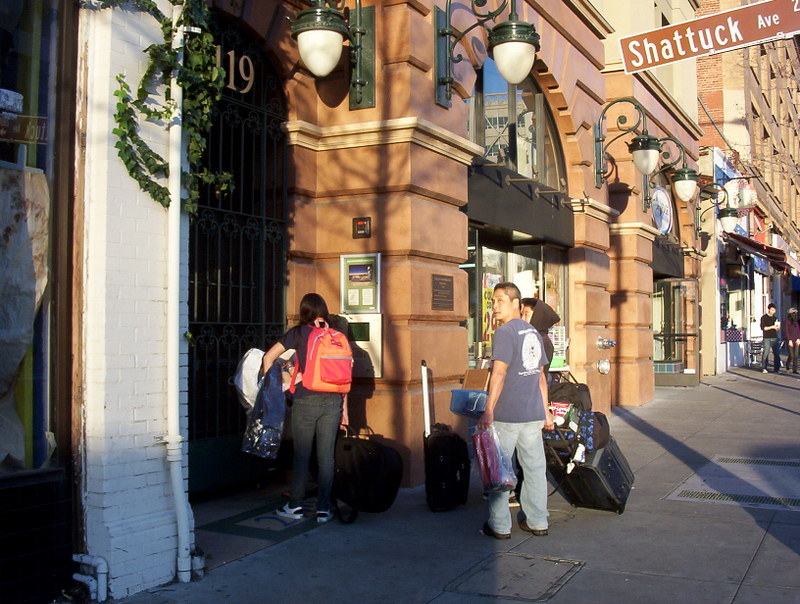The photograph captures a bustling sidewalk scene on Shattuck Avenue, with a well-maintained, light brown or beige building visible in the background. At the center of the image, three individuals are preparing to enter a building marked "119" in gold above the entrance. On the left side, we see the back of a person with dark hair, dressed in dark jeans and a dark shirt, carrying an orange backpack, a black suitcase, and a blue blanket. In the middle-right, a man in a blue shirt, also wearing jeans, glances back at the camera while holding a black suitcase in his right hand and a bag in his left. Further in the background, another person, partially visible, is dressed in a brown hoodie. The trio appears to be travelers, each laden with luggage. Additional people can be seen toward the right end of the image, standing on the well-kept gray sidewalk that runs parallel to several tall buildings stretching down the street. The bright, clear sunlight suggests a warm day, complementing the travelers’ casual attire.